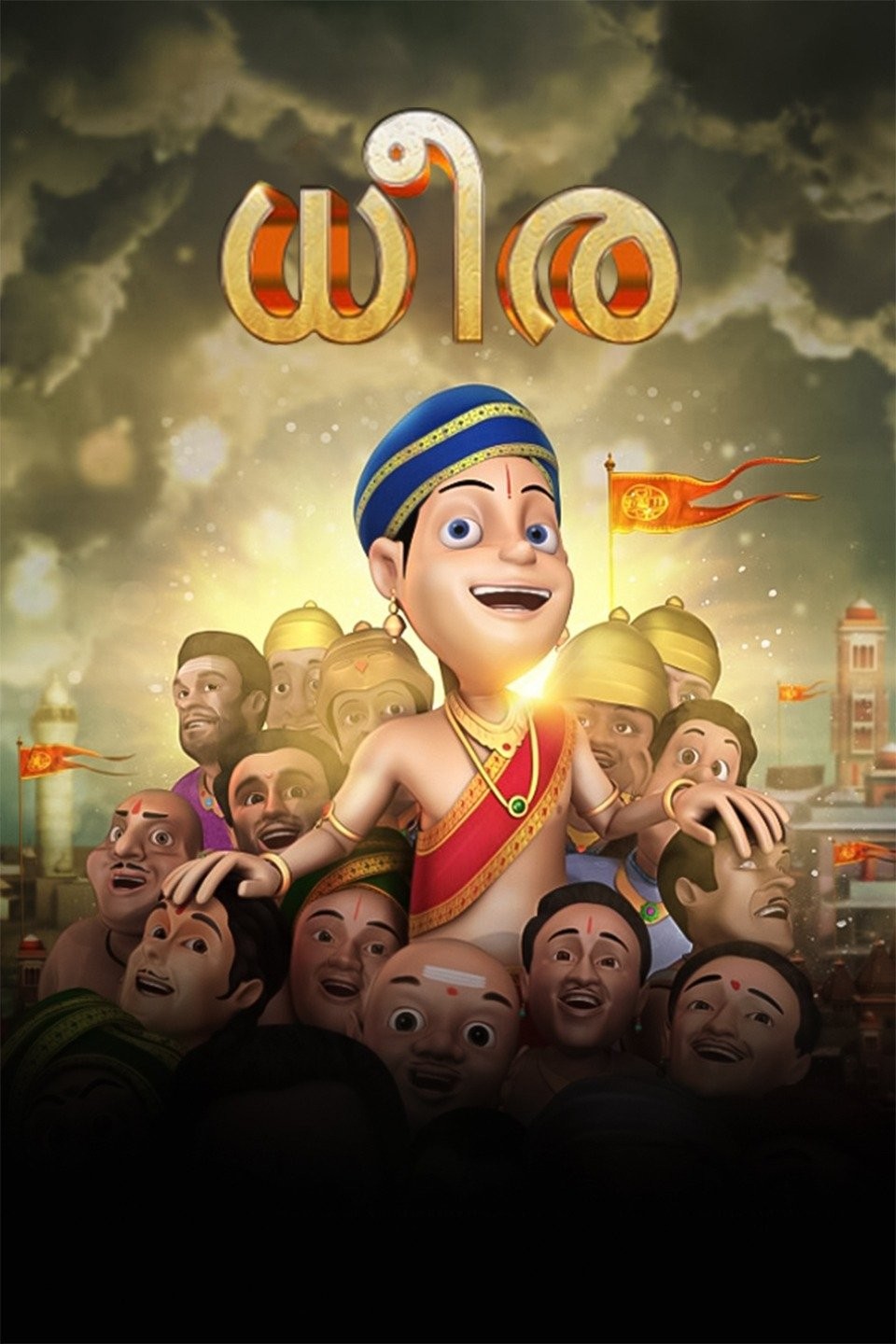This cartoon-style poster, likely for a video game, features an ensemble of animated male figures that appear to be of Middle Eastern or Indian descent. Dominating the center of the image is a larger-than-life character, distinguished by a blue and gold turban and a red sash draped across his chest, while he stands shirtless adorned with two gold necklaces—one snug with a red jewel and another looser with a green gem. With a dark sideburn peeking out and a small red vertical line between his eyebrows, his expressive face displays large eyes, a round nose, and a wide smile, accented by a golden bell-shaped earring in his right ear. His hands rest on the heads of two other men in the crowded foreground, suggesting his prominence. Surrounding him are multiple male figures, each marked on the forehead, including four individuals in gold helmets. One of these helmeted figures features a flag with a red banner and a golden logo. Above this vivid assembly of characters stretches a string of three-dimensional gold text in an unfamiliar script, likely the game's title. The urban background and dynamic composition suggest an adventurous or strategic narrative.